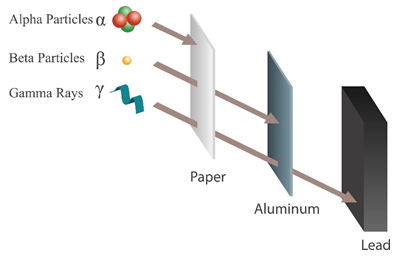This illustration, likely from a physics textbook, features a detailed diagram on a white background, showcasing the penetration abilities of different particles through varying materials. From left to right, three square plates of increasing thickness and decreasing height are aligned: the first is labeled 'paper' and is white, the second is labeled 'aluminum' and is a soft blue, and the third is labeled 'lead' and is black. The diagram is organized with descriptions on the left and corresponding images on the right. 

Starting with alpha particles, represented by a green jelly bean with red dots and labeled with a lowercase 'a', the diagram shows these particles being stopped by the paper plate. Next are beta particles, depicted as a yellow ball and marked with an uppercase 'B', which penetrate the paper but are stopped by the aluminum plate. Finally, gamma rays are illustrated by a blue ribbon-like wave and denoted with the Greek letter 'γ'. These gamma rays pass through both the paper and aluminum plates, only to be halted by the lead plate. Arrows illustrate the path and stopping points of each particle, providing a clear and educational visualization of particle penetration capabilities.